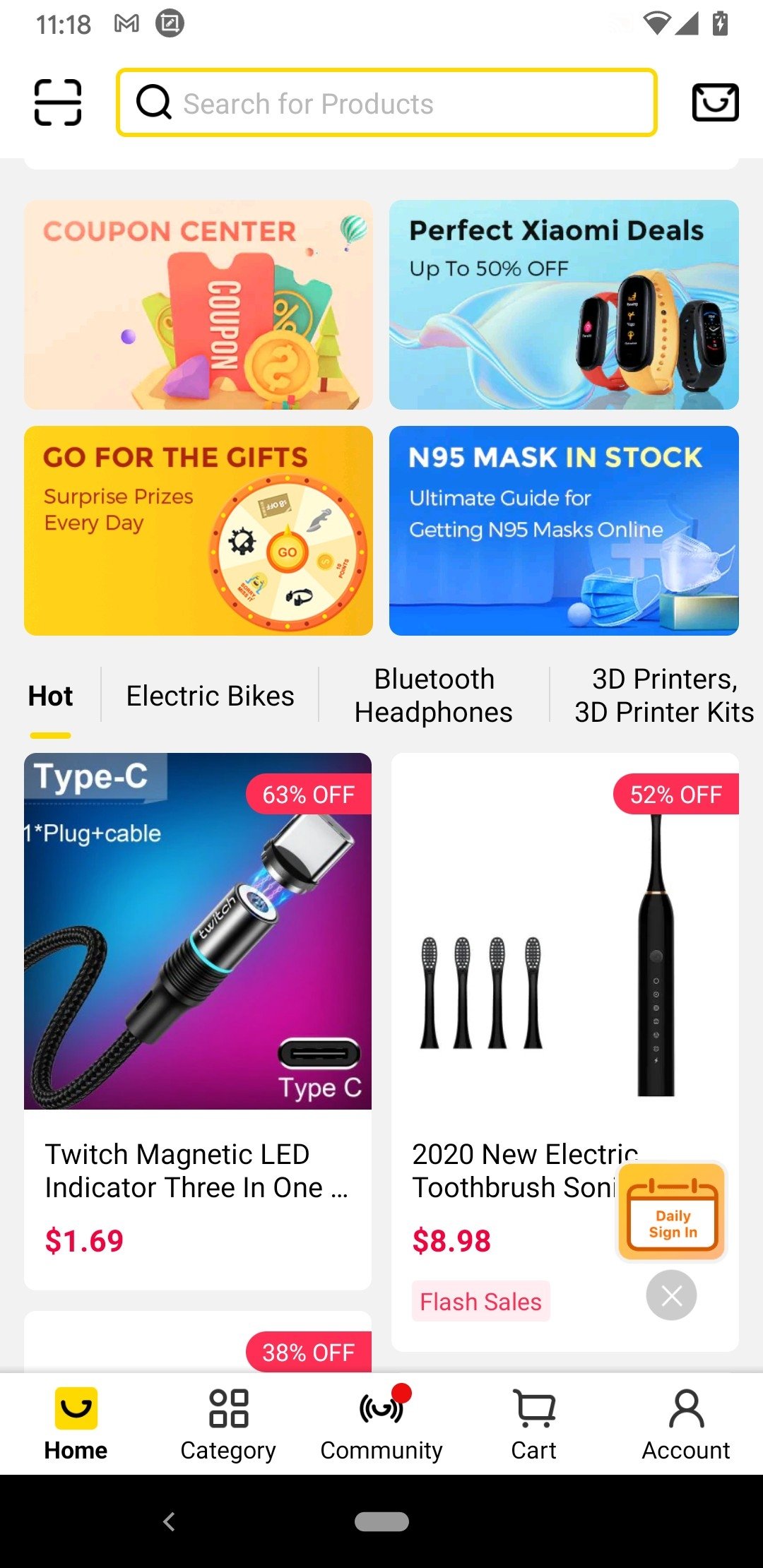This screenshot captures a mobile shopping application interface displayed on a phone. At the very top, there's a white header. Positioned left to right, the header contains dark grey text displaying "1118", followed by an "M" logo, and to its right, a grey circle with a white square inside. In the top right corner, there are three icons: a nearly full dark grey Wi-Fi icon, a full mobile signal icon resembling a triangle, and a mostly full battery icon containing a white lightning bolt.

Beneath the header, three elements are aligned horizontally:
1. On the left, there's a black icon resembling a set of corner shapes with a horizontal line through the middle, resembling a stylized square with a divider.
2. At the center, a white search bar outlined in yellow houses a dark grey magnifying glass icon on the left, followed by light grey placeholder text that reads "Search for products."
3. On the right, a dark grey envelope-shaped icon with a curved front.

The main body of the page features a light grey background with multiple tiles, each bearing different colored backgrounds, titles, and images:
- The top left tile has an orange title "Coupon Centre" with a clipart-style image of coupons below.
- The top right tile displays black text that reads "Perfect Xiaomi Deals, Up to 50% Off," accompanied by an image of fitness trackers to the bottom right.
- The bottom left tile features a caption "Go for the Gift, Surprise Prizes Every Day," alongside a clipart-style spinning luck wheel on the lower right.
- The bottom right tile, set against a blue background, states in white text, "N95 Mask in Stock, Ultimate Guide for Getting N95 Masks Online," with an image of two masks, one blue and one white, positioned at the bottom right.

Below these tiles, additional sections and product listings are visible.